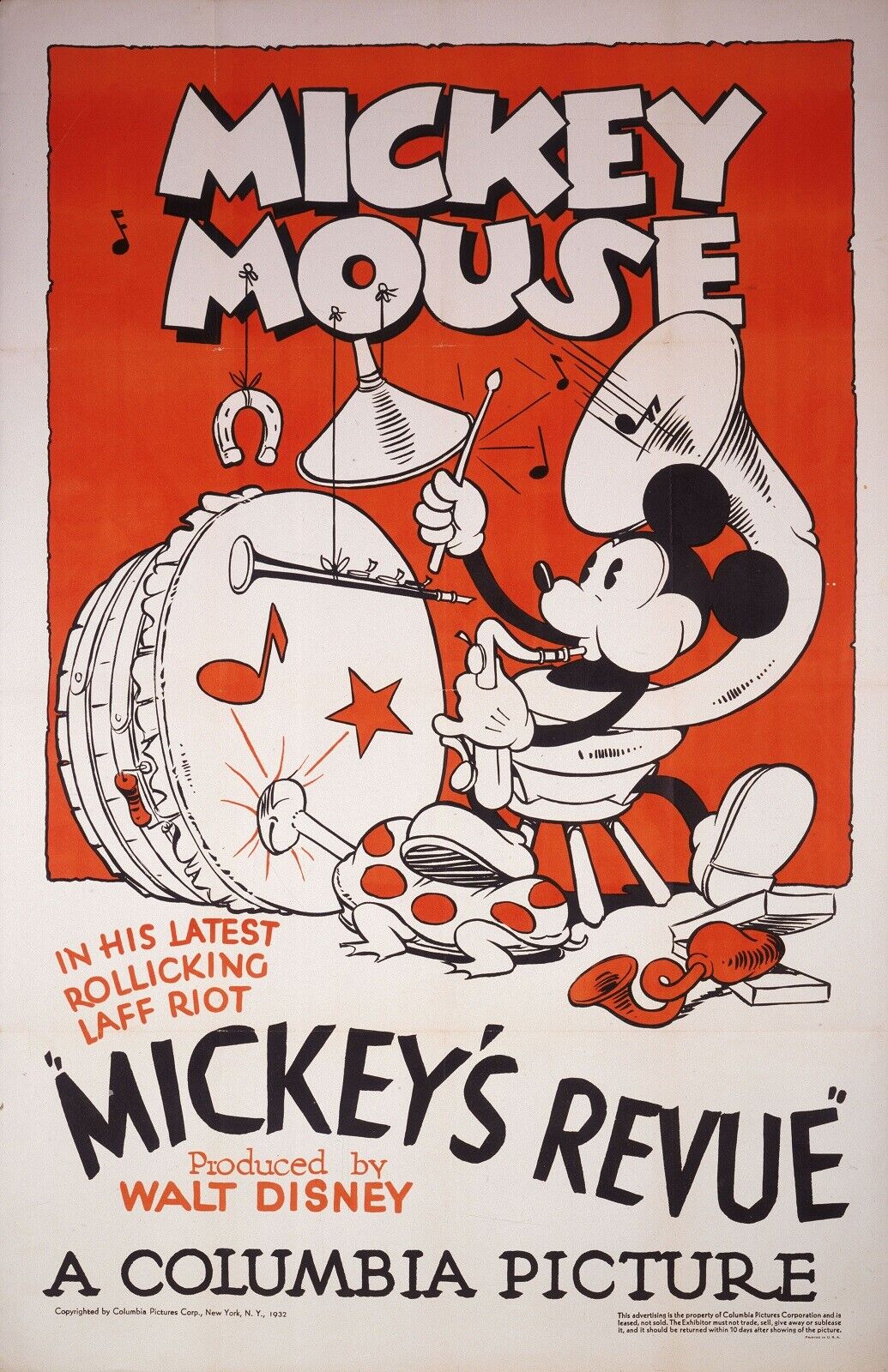This is an intricately detailed poster, either original or a reproduction, advertising the Mickey Mouse cartoon "Mickey's Review," produced by Walt Disney and distributed by Columbia Pictures. The vibrant color scheme consists of red, white, and black. At the top, large white letters outlined in black spell out "Mickey Mouse" against the red background, which extends slightly more than halfway down the poster before transitioning to white.

The central image features Mickey Mouse as a whimsical one-man band. He is depicted multitasking with delightful chaos: a saxophone is wrapped around his waist, he's beating a drum, clashing cymbals, and is seated on a stool. Both his feet are engaged in the act—one pressing down on an instrument and the other stepping on a turtle, which in turn hits the drum with its head. Mickey is also seen playing a tuba and a clarinet simultaneously, adding to the lively scene. Musical notes and a hanging horseshoe further enhance the lively atmosphere.

Below this animated illustration, in red letters, is the promotional slogan "In his latest Rollicking Laugh Riot." Beneath that, in bold black letters, is the title "Mickey's Review," followed by the credit "Produced by Walt Disney" in red, and finally "A Columbia Picture" in black letters. This poster, with its distinctive 1950s vibe, captures the essence of Mickey Mouse's vibrant and multifaceted character, promising an engaging and humorous cartoon experience.